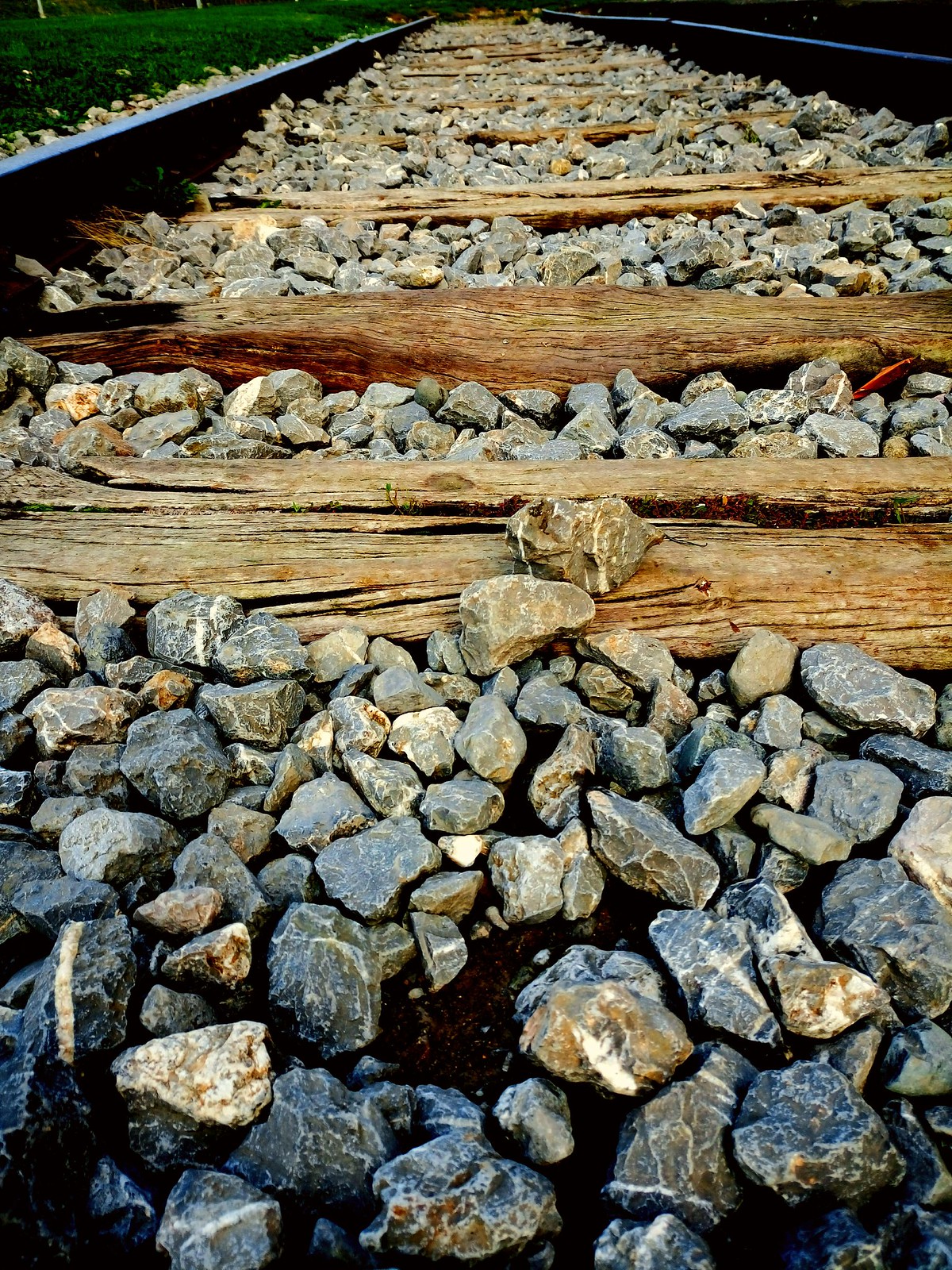The image offers a close-up perspective of railroad tracks captured from a low-angle ground view. Central to the composition, the parallel metal rails stretch away into the distance, visually converging at a single point. Interspersed between the rails are wooden railroad ties of light to medium brown color spaced evenly apart. The ground between the ties is covered in a mix of gray, brown, and white gravel and medium-sized stones, some of which spill over onto the wooden slats. Adding a layer of natural contrast, patches of green grass peek through on the top left corner of the picture, with some of the rocks dispersed along the edges by the grass. The detailed texture of the gravel and the weathered look of the wooden ties are prominent, reinforcing the sense of perspective as the eye follows the tracks into the distance.